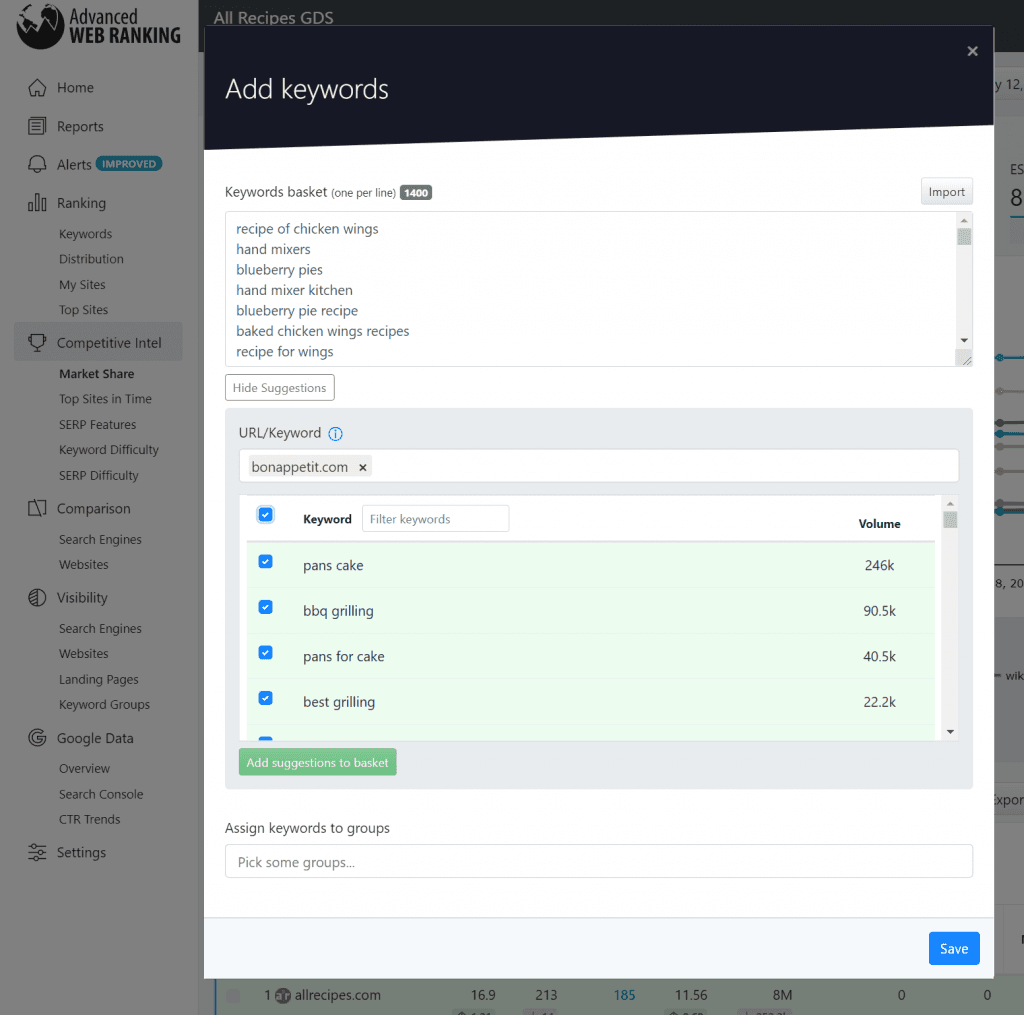This image depicts a detailed interface of a web page related to SEO and keyword ranking tools. The left sidebar has a gray background and prominently features the heading "Advanced Web Ranking" at the top, accompanied by a globe icon. Below this, several menu items are listed:

1. Home (with a Home icon)
2. Reports (with a piece of paper icon)
3. Alerts (with a bell icon)
4. Ranking (with a bar graph icon)

Sub-items under "Ranking" include:
- Keywords
- Distribution
- My Sites
- Top Sites

Next, a highlighted section reads "Competitive Intel" with a cup-like icon adjacent to it. Under this, the submenu items are:
- Market Share
- Top Sites and Times
- SERP Features
- Keyword Difficulty
- SERP Difficulty

Below "Competitive Intel," another section titled "Comparison" lists:
- Search Engines
- Websites

Then, the "Visibility" section includes:
- Search Engines
- Websites
- Landing Pages
- Keyword Groups

Further down, a category labeled with a G icon, "Google Data," encompasses:
- Overview
- Search Console
- C2R Trends

Finally, the last item on the sidebar is "Settings."

The larger central panel of the web page starts with the header "Add Keywords." Here, there are sections for keyword entry and management. The first section is titled "Keywords Basket" (one per line), indicating the entry of 1,400 keywords such as "Recipe of Chicken Wings," "Hand Mixers," "Blueberry Pies," "Hand Mixer Chicken," "Blueberry Pie Recipe," "Baked Chicken Wings Recipe," and "Recipe for Wings."

The next section titled "URL Keyword" contains a search bar pre-filled with "bonappetit.com." Below this, filters are applied to keywords, listing them in blue squares with checkmarks, including "Pan's Cake," "BBQ Grilling," "Pans for Cake," and "Best Grilling."

At the bottom of the panel, there is an option to "Assign Keywords to Groups," featuring a white input rectangle for further keyword organization.